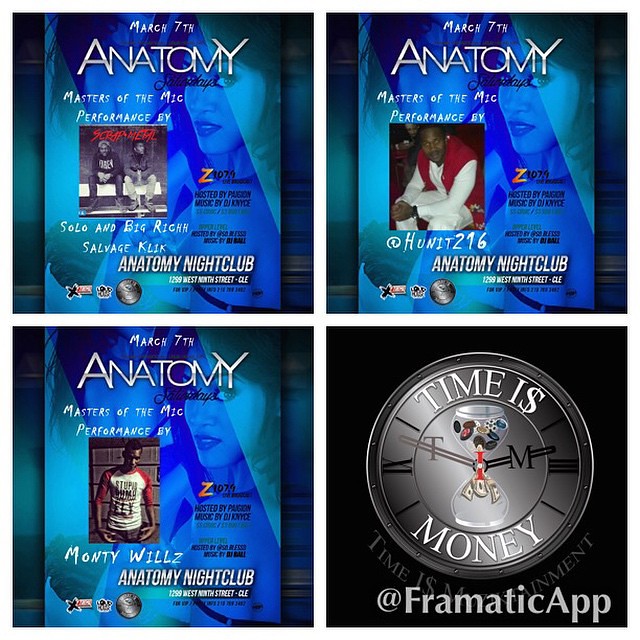This image is an advertisement for Anatomy Nightclub, divided into four equal quadrants. The top three quadrants feature a blue background with a faded image of a woman on the right half. Each of these quadrants promotes a different artist set to perform on March 7th under the "Masters of the Mic" event title. The top left quadrant shows two men sitting on a bench, labeled "Solo and Big Rich Salvage Clique." The top right quadrant features a single man with the title "Hunt 216 Performer." The bottom left quadrant presents another man, identified as "Monty Wills." Each promotion includes gray, capitalized text saying "Anatomy Nightclub" at the bottom.

The bottom right quadrant diverges from the others with its black background and a distinctive image of a clock face. Instead of hour numbers, the clock reads "Time is Money," with an hourglass at its center. Below this, it says "At Chromatic App," indicating some form of affiliation or partnership. The entire poster is predominantly aqua and blue in color, maintaining a cohesive aesthetic.